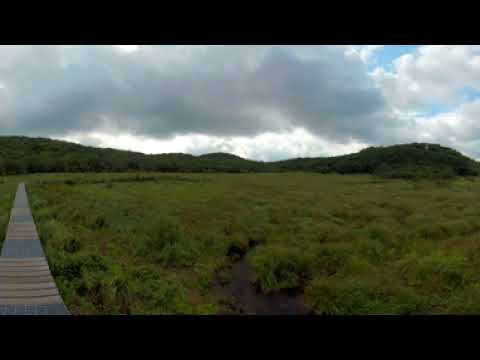This image portrays a serene outdoor landscape dominated by lush greenery and a wooden boardwalk. The boardwalk, composed of wooden planks, starts at the bottom left corner of the image and stretches into the distance, gradually narrowing as it approaches the horizon. It runs parallel to a vast, grassy expanse on the right side of the image. The grass appears dense and lush, interspersed with occasional marshy patches where water peeks through the vegetation.

In the background, a range of low-lying hills or ridgelines extends across the entire width of the photo. These hills are adorned with a mixture of darker green foliage, likely composed of grass, bushes, and possibly some low vegetation, though they are not very tall or mountainous.

Above the landscape, the sky is predominantly covered with thick clouds, adding a sense of impending weather change or moisture in the air. The cloud cover is denser and darker towards the left side of the image, suggesting a potential storm, while the right side shows lighter, more wispy clouds and a small patch of blue sky peeking through. The sun also makes a subtle appearance through these clouds, casting a gentle light over the scene.

Overall, the image captures a tranquil, green-dominated outdoor setting with a sense of depth and natural beauty, framed by a thick black border at the top and bottom.